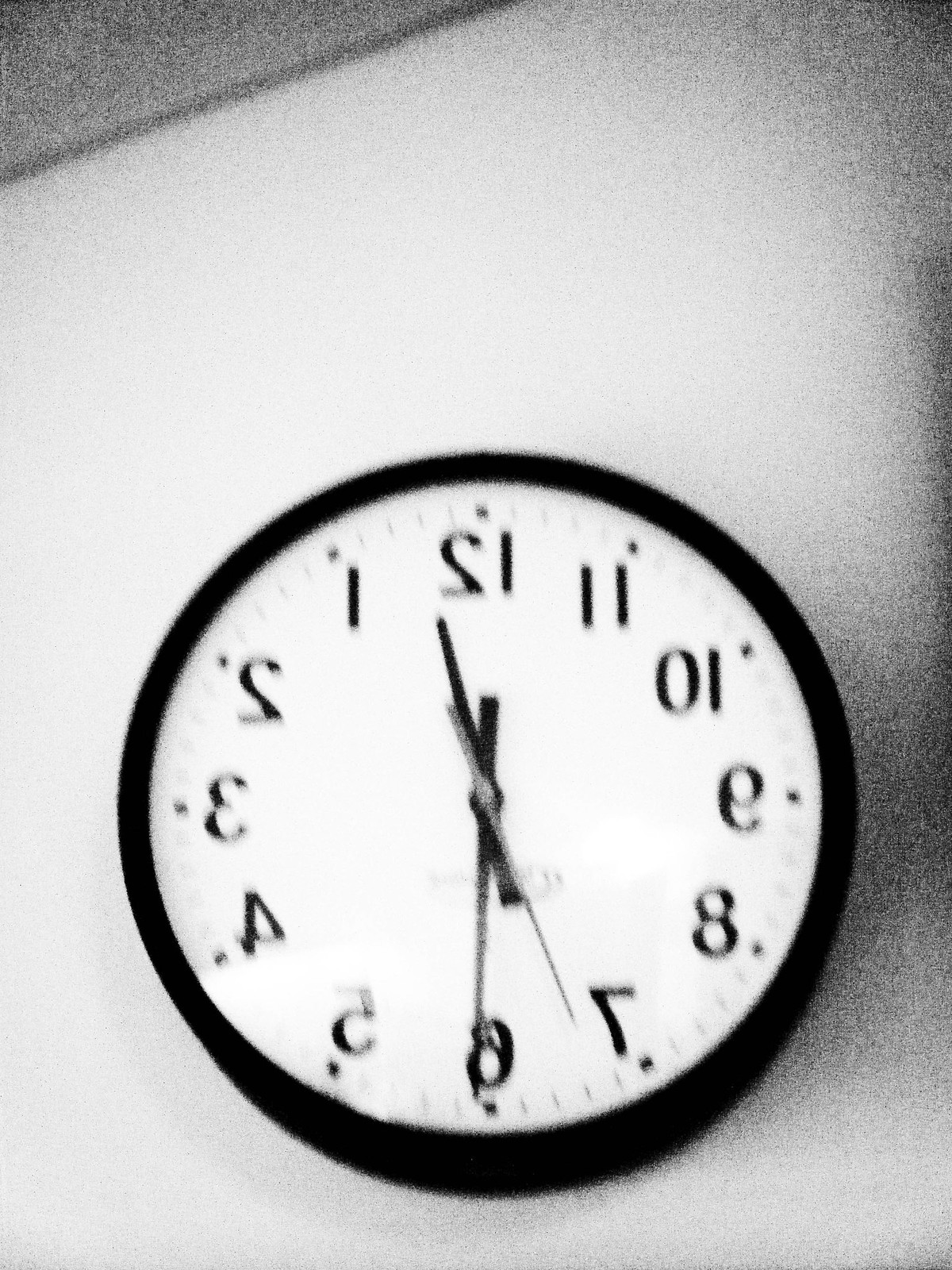This black and white photograph features a wall clock displayed in reverse, creating a mirror image effect where all the numbers appear flipped. The clock is mounted on a white wall and its thick, black frame, likely made of plastic, contrasts starkly against the background. The clock face is white, adorned with numerals that have a slight calligraphy flair. The clock’s hands are slender and pointed. Notably, the right side of the image is heavily shadowed and exhibits significant graininess, adding a distinct, textured quality to the photo.